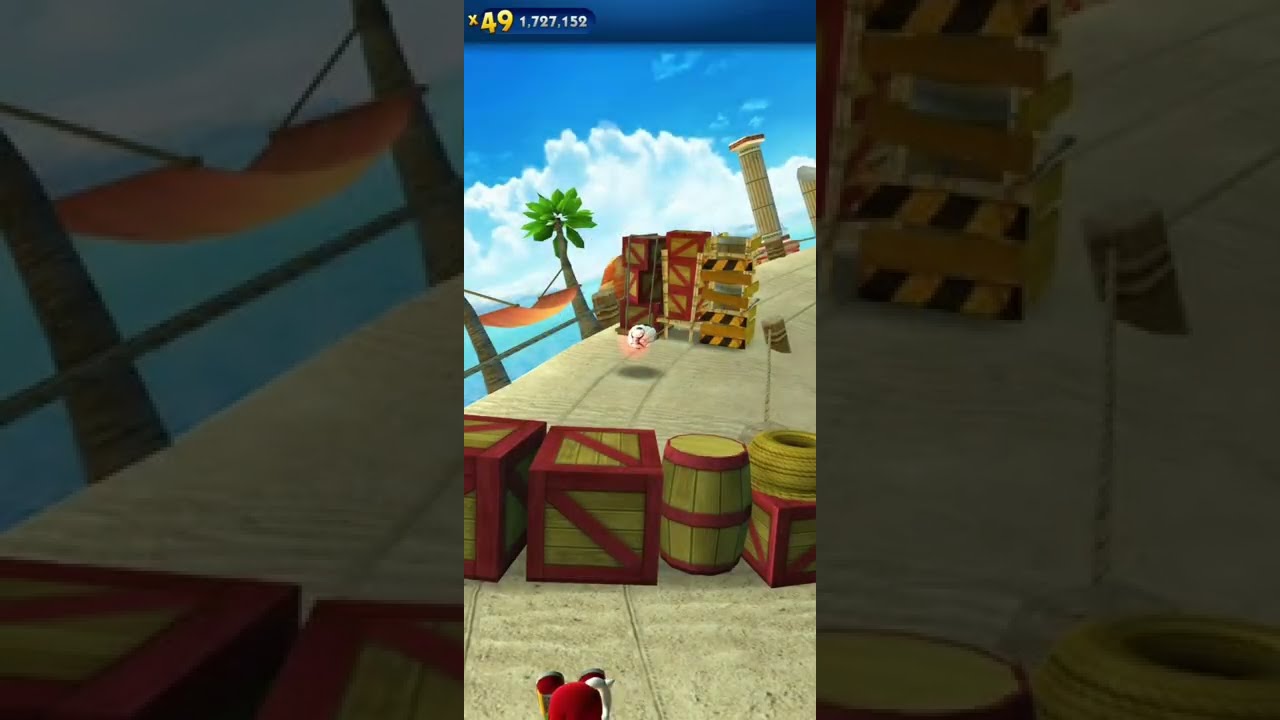This high-definition image is divided into three distinct panels, with the central panel being the most prominent and the brightest, resembling the shape of a smartphone screen. It appears to be a still from a vibrant, tropical-themed video game, showcasing a dock area brimming with details. In the central panel, a stone dock is flanked by two soaring palm trees holding up a hammock, creating a paradisal setting. The dock is cluttered with wooden crates and barrels outlined in red, suggesting a loading area. Some of these crates are closer, while others recede into the background, adding depth to the scene.

Above this illustration, a dark blue header spans the top of the image, displaying a gold “X 49” and the number “1,727,152” in white. The floor of the dock appears brown and segmented into multiple lanes, hinting at a running track where crates and barrels may need to be jumped over or broken through.

In the background, a serene blue sky riddled with cumulus clouds stretches overhead, occasionally punctuated by tall trees and Greco-Roman style columns. Completing the scene are eye-catching yellow and black diagonal road signs marked "don't enter," adding an element of caution amidst the idyllic setting. The left and right panels, more faded and darker, feature close-ups of items from the central image, specifically the hammock on the left and one of the crates on the right, replicating parts of this lively illustration and enhancing the depth and immersion of the central panel.